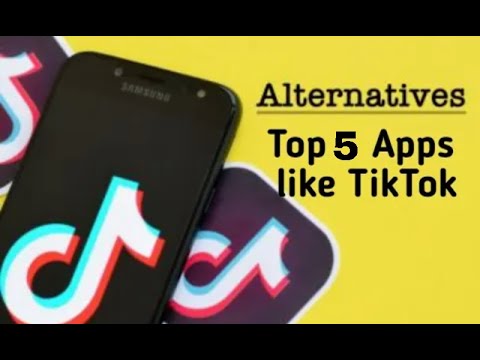Screen capture of a website header or advertisement for an article titled "Alternatives: Top 5 Apps Like TikTok." The layout features a bright lemon yellow background with contrasting black text. The word "Alternatives" is underlined, drawing attention to the focus of the content. The header includes a black stripe at both the top and bottom, adding a letterbox effect. On the left side of the image is a black Samsung phone displaying the TikTok logo on its screen. In the background, multiple TikTok icons are superimposed, each featuring the familiar black backdrop with the TikTok symbol outlined in light blue and red, all encased in a white border.